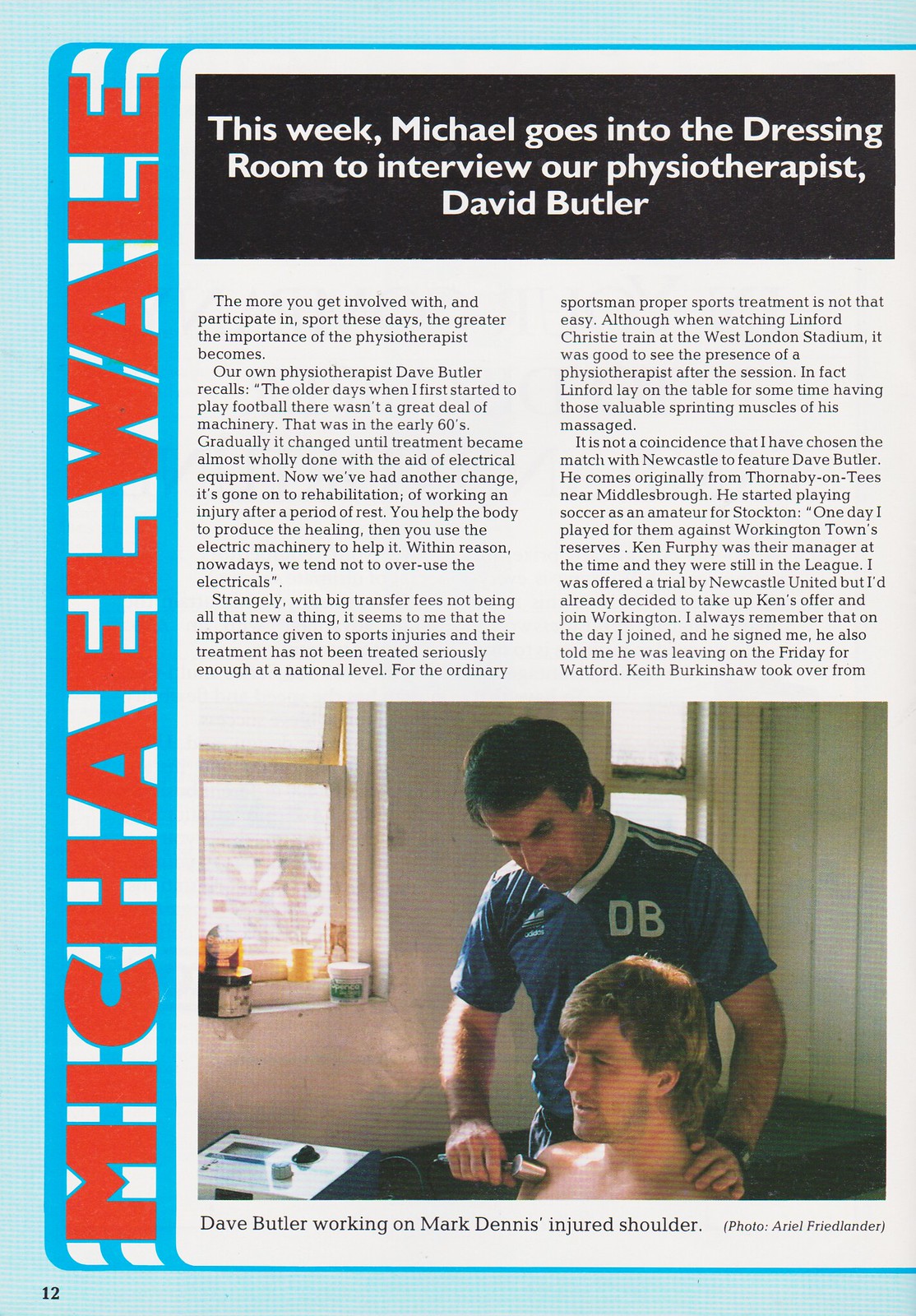The image is a detailed color scan of page 12 from a Match Day program promoting an English soccer game. The page is predominantly white with a light blue top edge, and a large red and blue vertical design on the left side, prominently displaying the name "Michael Whale." At the top center, in a black box with white text, it reads, "This week Michael goes into the dressing room to interview our Physiotherapist David Butler."

The main feature of the page is a photograph at the bottom showing two men in a dressing room. One man, likely Mark Dennis, is shirtless and sitting down, while another man, identified as Dave Butler, stands behind him wearing a blue short-sleeved shirt with "DB" printed on it. Dave Butler is using a medical device on the sitting man's right shoulder. The caption under the photograph states, "Dave Butler works on Mark Dennis' injured shoulder," and credits the photographer, Ariel Friedlander.

The accompanying article dives into the role and importance of physiotherapy in soccer. It recounts Dave Butler's career journey from playing amateur soccer to becoming a physiotherapist, emphasizing the evolution of sports treatment from minimal equipment in the 1960s to modern-day rehabilitation technologies. The text highlights Butler’s significant role in the team's healthcare, reflecting on historical changes in sports medicine and its critical impact on athletes' performance and recovery.